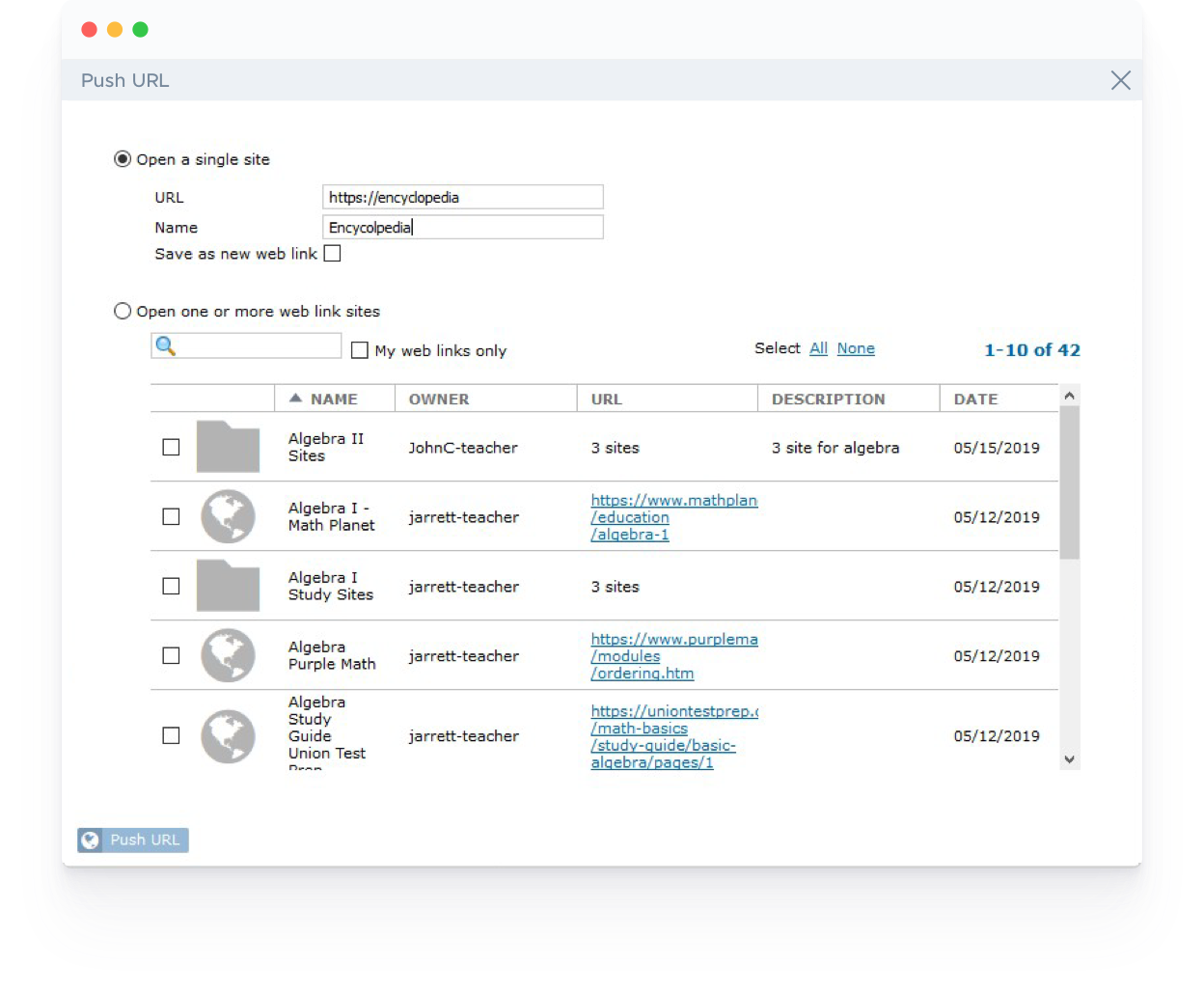The image showcases a user interface with various elements and sections, each described in meticulous detail:

At the top left corner, there is a light gray header with a distinctive red circle, followed by a yellow circle, and then a green circle. Below this, a slightly darker gray border contains the text "push URL" in black on the left side, and a black "X" on the right side.

The main section features a clean, white background. Directly under the gray border, there is a black circle with a white border, which is described as "open a single site." Next to this, to the right, it says "URL" with a text box to enter a URL, and then "Name" followed by another text box for entering a name. Below this section, the interface offers the option "save as a new web link," accompanied by a white square with a black border. Beneath these elements, there is another circular white button with a black border that says "open one or more web links." Following this is a search bar, a square with possibly a function icon, and the text "my web links only" to the right of it.

Toward the middle right side of the interface, there is text that says "Select" in black, then "All" in blue and underlined, and "None" in blue and underlined. Below this selection, there is an indication of "1-10 of 42." 

The section beneath features a row with five columns: the first being empty, followed by "Name," "Owner," "URL," "Description," and "Date," all within a gray bar. 

Within the leftmost column, under the empty section, there are smaller squares, each featuring a black border with alternating file and globe icons stacked from top to bottom.

In the columns under the "Name," "Owner," "URL," "Description," and "Date" headings, respective information about the sites, teachers, URLs, descriptions, and dates are displayed.

In the bottom left corner, there is a blue tab that reads "push URL" in white text.